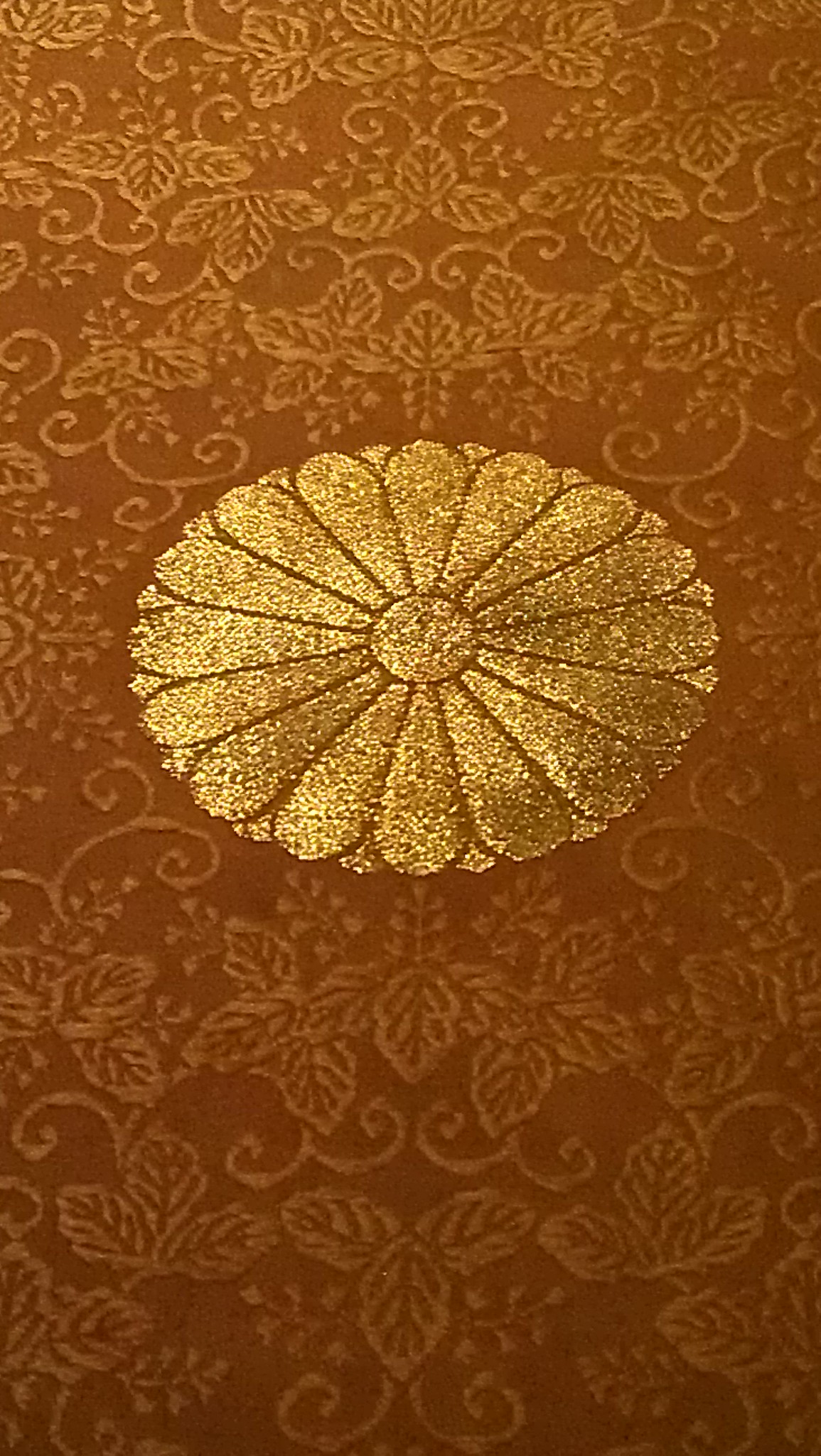This image features a close-up of an ornate decoration that could be part of a tablecloth, curtain, or rug, primarily set against a brown gradient background that transitions from light to dark from top to bottom. The central focus of the image is a large, shimmering gold flower, resembling a sunflower, with teardrop-shaped petals arranged in a 360-degree pattern around a circular center. The flower is detailed with golden sparkles, making it the prominent element of the design. Surrounding the central flower are various golden plant-like patterns, including leaves and possible pinecones, adorned with intricate squiggly lines and swirls. The harmonious interplay of these elements creates an elaborate and luxurious pattern that embellishes the brown and gold backdrop, suggesting a sophisticated and decorative fabric piece.